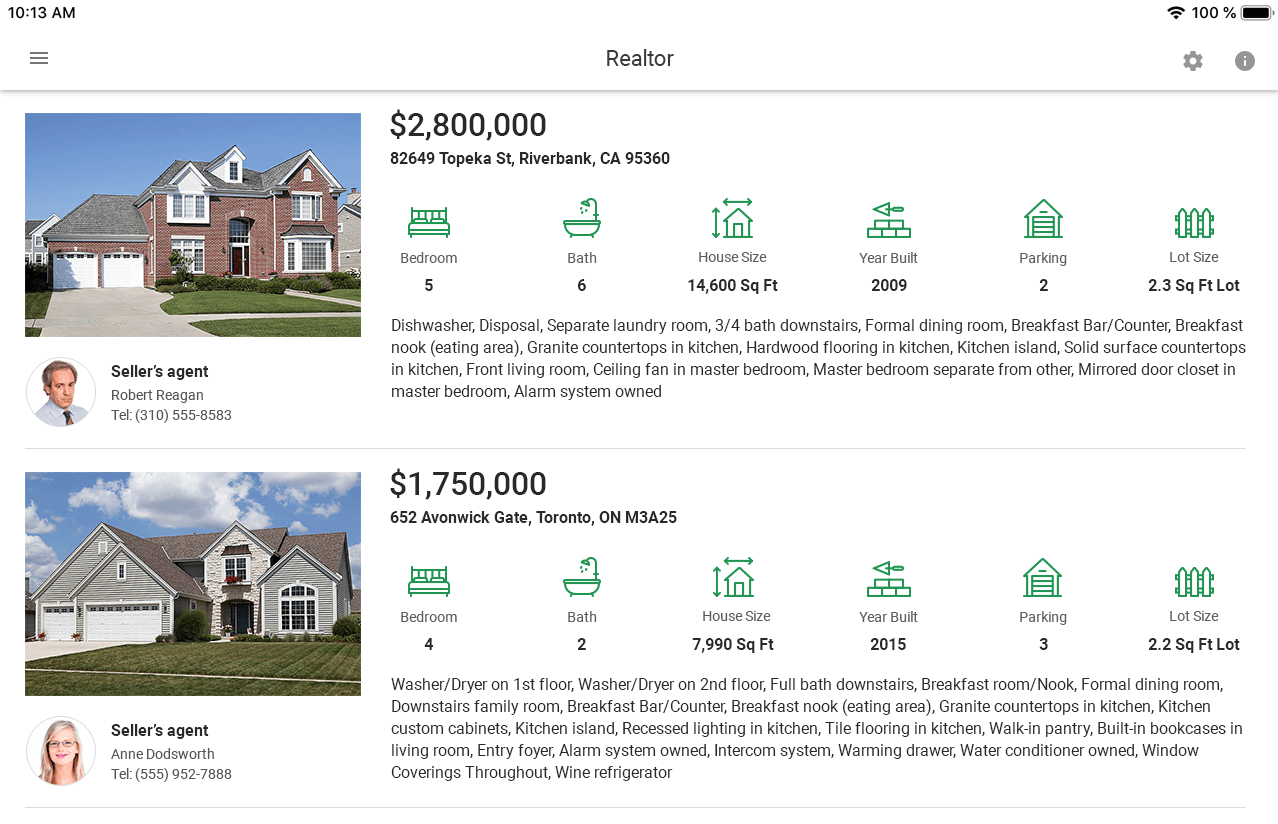This screenshot depicts listings from a real estate page set against a white background. The image was captured at 10:13 a.m. and shows a fully charged battery in the top right-hand corner. The word "Realtor" is prominently displayed in the middle of the screen, with a gray line running horizontally across the page.

The first listing highlights a luxurious property priced at $2.8 million, located at 82649 Topeka Street, Overbank, California, 95360. This expansive home, built in 2009, encompasses 14,600 square feet and sits on a 2.3-acre lot. It boasts five bedrooms and six bathrooms. Notable features include:
- Two-car garage
- Dishwasher and disposal
- Separate laundry room
- Three-quarter bath on the ground floor
- Formal dining room
- Breakfast bar, counter, and nook
- Granite countertops in the kitchen
- Hardwood flooring in the kitchen
- Kitchen island and solid surface countertops
- Front living room
- Ceiling fan in the master bedroom
- Master bedroom separate from other rooms
- Mirrored closet doors in the master bedroom
- Owned alarm system

The second listing is for a more recent home valued at $1.75 million, situated at 652 Avenue Gate, Toronto, Ontario, M3B 825. This property, built in 2015, features:
- Four bedrooms and two bathrooms
- A total area of 7,990 square feet
- Three-car garage
- 2.2-acre lot
- The seller's agent is named Ann Doddsworth, contactable at (555) 952-7888.